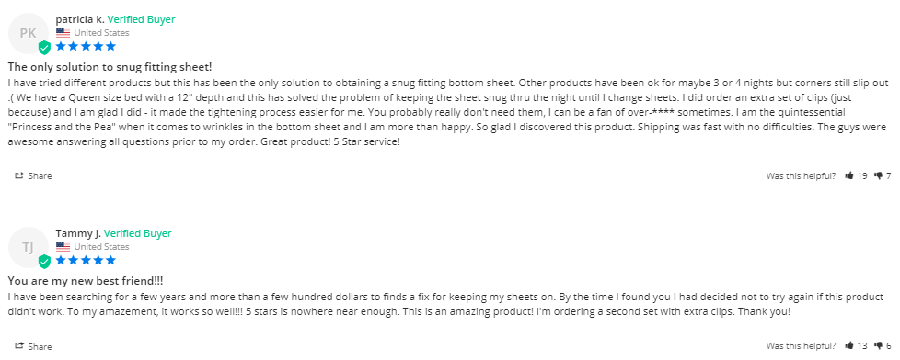This screenshot showcases two detailed customer reviews from my website against a sleek, white background.

At the top left, there's a light gray circular icon containing the initials "PK." Next to it, the name "Patricia K." is displayed in lowercase letters, followed by the term "verified buyer" in green. Below, there's an American flag icon with the label "United States." Patricia gave a five-star rating in blue, accompanied by a green shield featuring a white checkmark, indicating buyer verification.

Patricia's review is titled, "The Only Solution to Snug-Fitting Sheets." She explains how she has tried various products to keep her bottom sheet snug, but this product has been the only effective solution. Despite other products failing within three or four nights, this product has successfully kept the sheets in place on her 12-inch deep queen-size bed. She also mentions ordering an extra set of clips, which made the tightening process easier, although not necessary. Patricia humorously refers to herself as the "quintessential princess and the pea" regarding wrinkles in the bottom sheet and expresses her satisfaction with the product, praising the fast shipping and excellent customer service. She concludes her review with a five-star rating in blue.

Below Patricia's review, there is another circular icon with the initials "TJ," followed by the name "Tammy J." with capitalized initials. Tammy is also a "verified buyer" from the United States and has provided a five-star rating in blue, along with the green shield indicating verification.

Tammy's review is titled, "You Are My New Best Friend." She recounts her long search over several years and countless products to keep her sheets in place. Upon discovering this product, she was initially skeptical but was amazed by its effectiveness. She enthusiastically states that five stars are insufficient to rate the product and plans to order a second set with extra clips. Tammy concludes with heartfelt thanks.

Both reviews highlight exceptional satisfaction with the product and commend the overall buying experience.